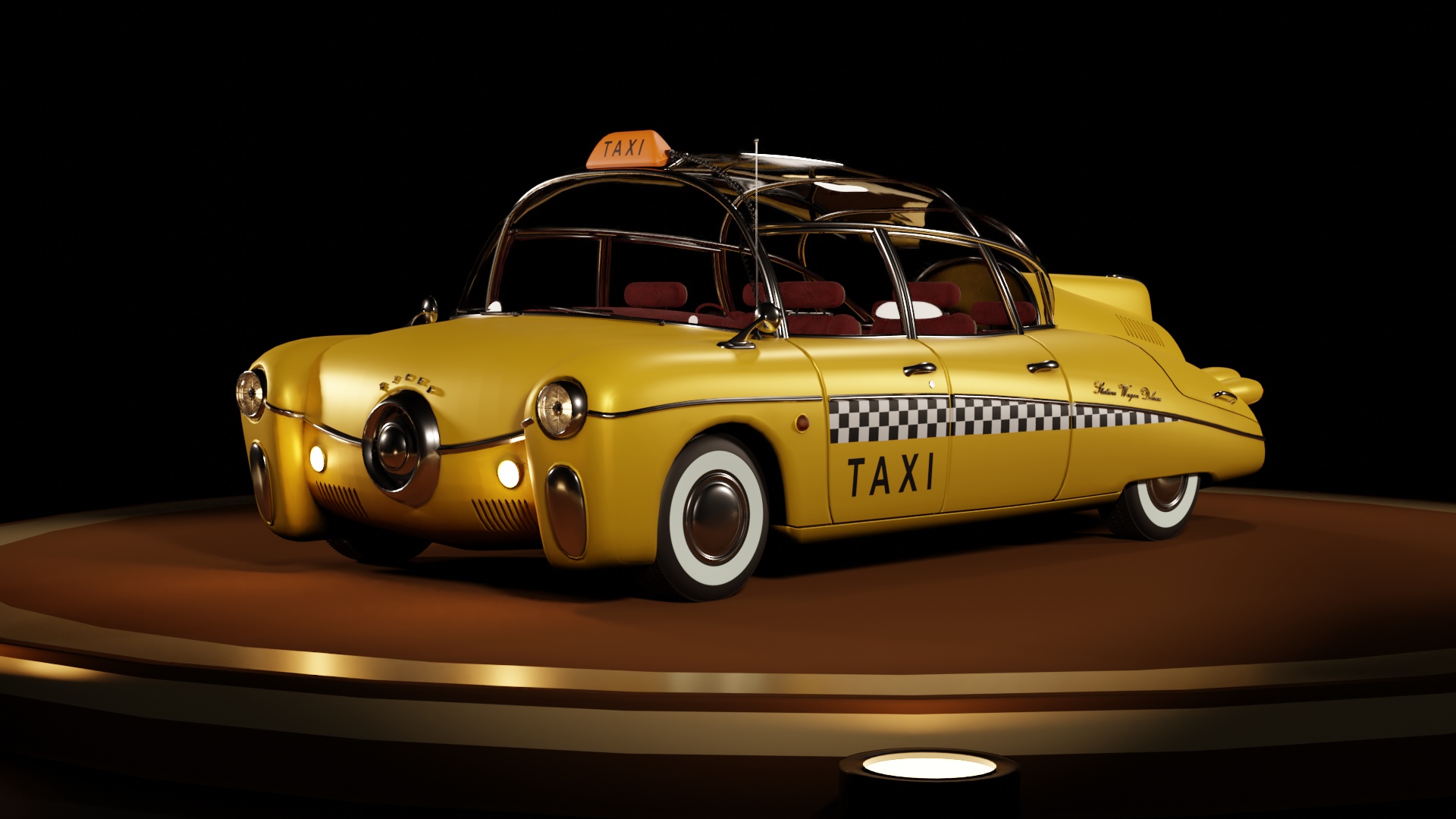The image depicts a detailed 3D model of a yellow toy taxi, positioned on a round, brown platform adorned with a gold ring and area lights. The taxi is oriented with its front on the left side of the frame, slightly angled forward, showcasing both the front and left side. The body of the taxi, resembling a submarine with wheels, features black and white checkered designs starting from the front door and tapering off towards the rear. Above this design, on the driver's door, is the word "TAXI" in black letters. The taxi has white wall tires and red seats in the interior. The roof is black, supported by bars instead of a solid windshield, and features window panels that extend down to the yellow body. On the yellow hood, the word "DODGE" is faintly visible above a round silver grille with headlights on either side and two oval lights on the lower fender. At the top, there's an orange taxi sign with black letters, paired with an antenna on the left side and windshield wipers. The entire scene is set against a black background, making the intricate details of the model stand out vividly.